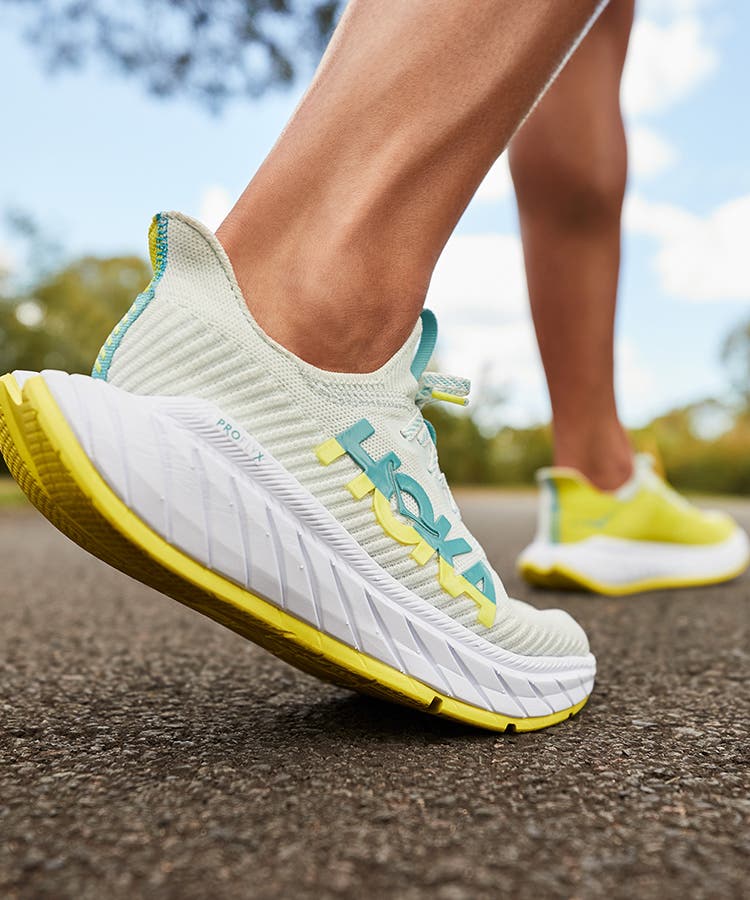The photograph captures a close-up view of a woman's lower legs and ankles, showcasing her defined and athletic build. She is wearing a pair of striking Hoka sneakers, prominently labeled "H-O-K-A" in capital letters with a unique logo in the 'O'. The Hoka lettering features a gradient, transitioning from teal on the upper half to yellow on the bottom half. The sneakers are primarily white with a thick sole that extends backwards and slightly curves up, potentially enhancing walking comfort. Detailed yellow accents appear on the sole and sides, and there are subtle touches of blue on the shoe's lip and the inner side. The shoelaces are mostly white with hints of yellow. The photo has an artistic focus on the footwear and the woman's poised tiptoes stance, with a blurred background revealing hints of blue sky, clouds, and greenery, all contrasting with the asphalt ground she's standing on.